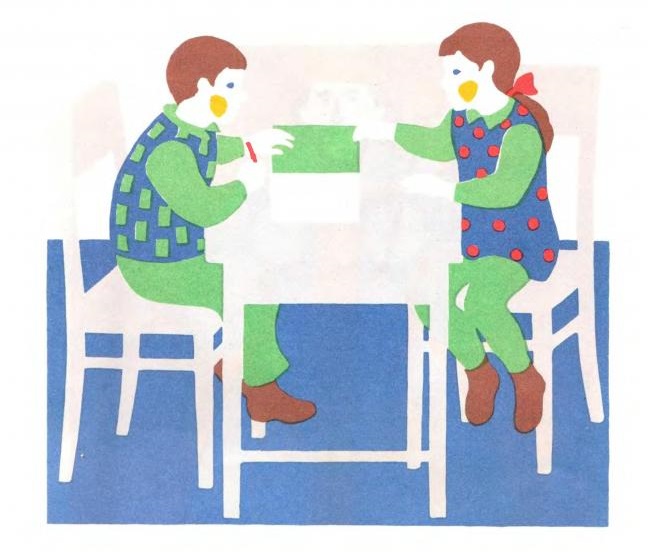The image is a simple, cartoonish child’s illustration depicting two children seated at a white table, set against a white background with a blue floor. The children are a boy on the left and a girl on the right. Both have brown hair and blue eyes, with distinct yellow spots painted on their cheeks. 

The girl has long brown hair adorned with a ribbon, and she is dressed in a green shirt and pants, a blue-and-red polka dot jumper, and brown shoes. The boy, sitting opposite her, wears a blue and green checkered vest, a green shirt and pants, and brown shoes. They are both leaning slightly forward, their hands resting on the white table. The detail of their white hands blends into the table, although the boy's hand appears to be holding a brown pencil.

Central to the image is the table and the chairs, which are also white. The children's legs are not touching the floor, indicating a playful, relaxed posture. They are both engrossed in what appears to be a green object, possibly a notebook, placed in front of them on the table, their gazes fixed intently upon it.